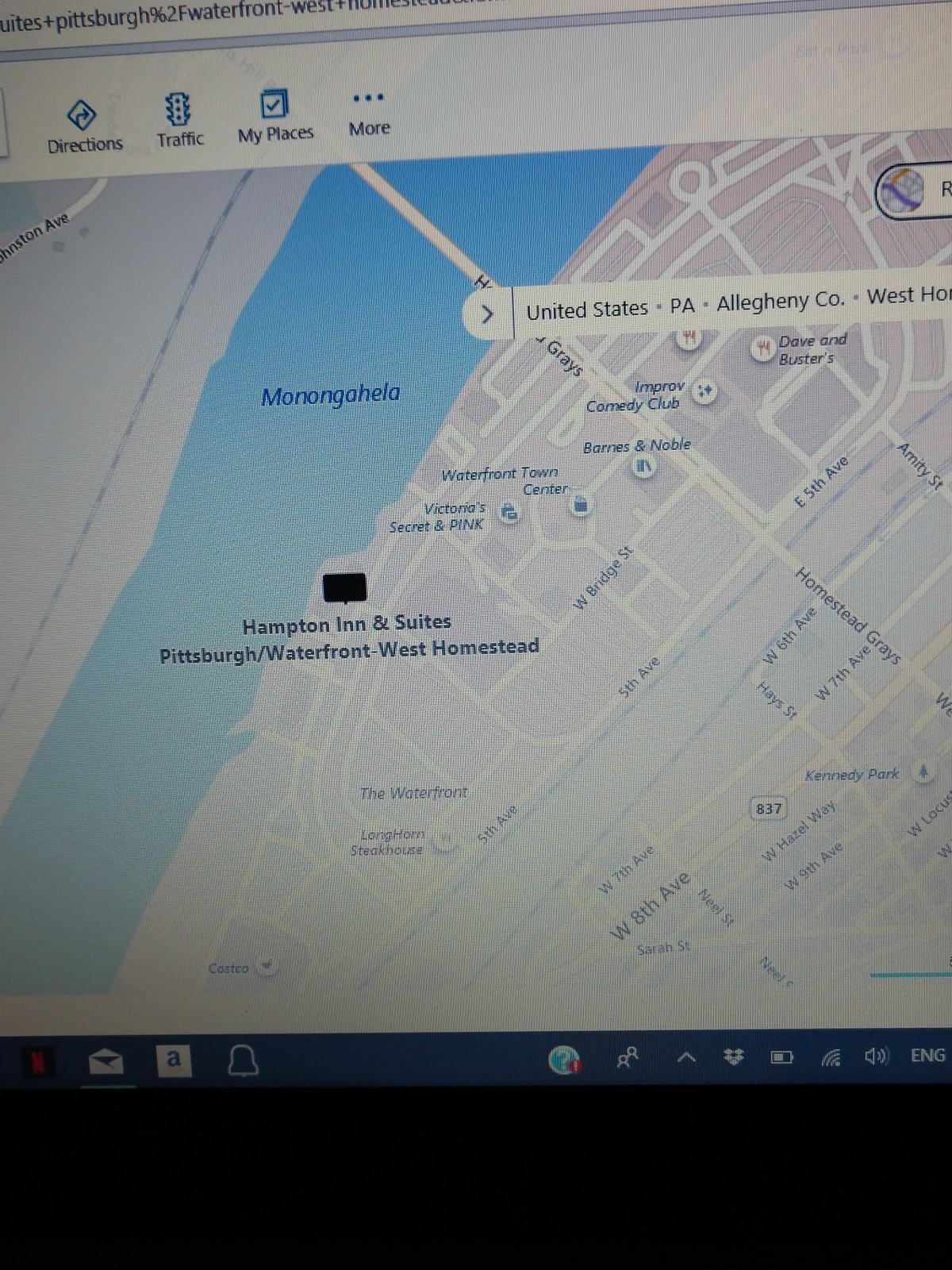The image is a photograph of a Windows computer screen displaying a navigation map of the United States, specifically highlighting Pennsylvania and Allegheny County. The map prominently features the Hampton Inn and Suites, Pittsburgh Waterfront West Homestead. Various surrounding towns, cross streets, and landmarks such as a Barnes and Noble, Waterfront Town Center, Victoria's Secret, and Dave and Buster's are visible. A notable geographical feature is the Monongahela River, labeled in blue, with a bridge connecting different parts of the area. At the top of the screen, navigation buttons labeled "Directions," "Traffic," "My Places," and "More" are visible. The screen also includes minor icons typical of a Windows interface at the bottom, further confirming the location and details of the map.